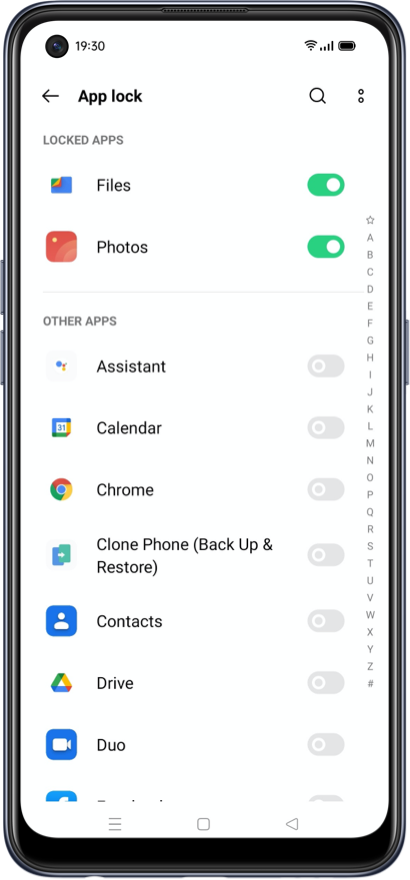This image depicts a smartphone with a distinct black and gray border. The device screen showcases a white background. At the top left corner, the time is displayed as 19:30, and to the right, a fully charged battery icon is visible. Below the status bar, there is a left-facing arrow icon labeled 'App Lock'. Below that, a list of app sections is presented, starting with 'Locked Apps', followed by 'Files' and 'Photos', both of which are highlighted or selected.

Further down, additional app categories are listed under 'Other Apps', each accompanied by on/off indicators. These apps include:
- Assistant (turned off)
- Calendar (turned off)
- Chrome (turned off)
- Clone Phone, Backup, and Restore (turned off)
- Contacts (turned off)
- Drive (turned off)
- Duo (turned off)

On the right-hand side of the screen, an alphabetical index is displayed, with each letter of the alphabet occupying a separate line vertically.